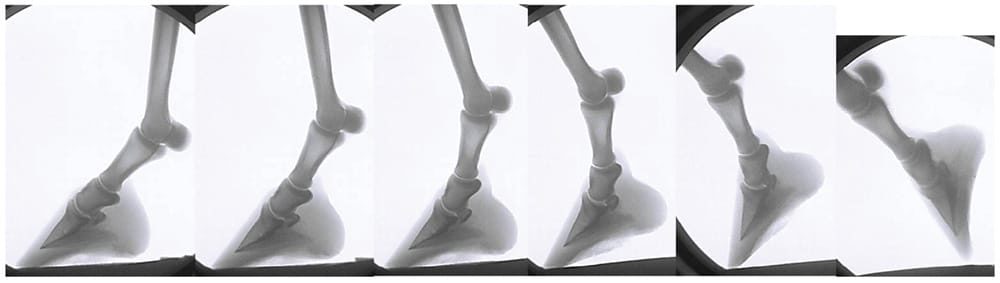The image features a series of six black-and-white depictions of a skeletal structure resembling an insect leg, presented in an x-ray style. Each close-up shows the leg in varying positions, progressing from a flat stance on the leftmost image to being up on its pointed tip in the rightmost image, suggesting a walking motion. The leg consists of sections that resemble bones, and it extends from the top of each frame, bending at an obtuse angle and tapering to a sharp, pointed end. The surrounding flesh, although indistinct, can be inferred from the shape, giving a sense of movement as if the leg is stepping forward. Despite the detailed and bone-like appearance, this might actually be a stylized painting or drawing.